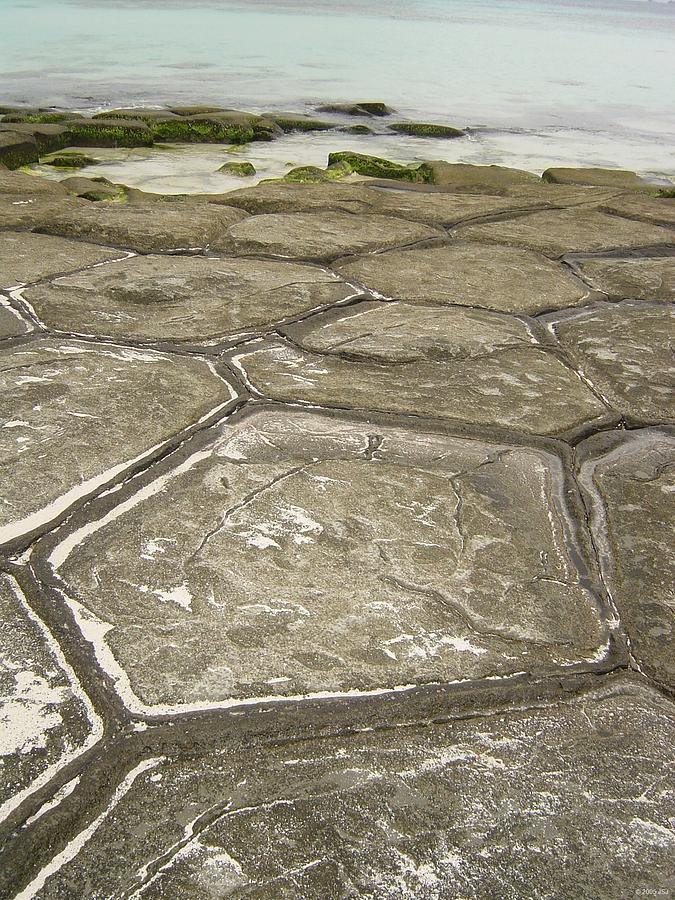The photograph captures a striking view of the ocean meeting the shoreline under daylight. The blue ocean, with waves visible in the distance, contrasts beautifully with a unique natural rock formation that resembles an intricately tiled floor. The rocks have shapes akin to a turtle's shell, featuring brown borders and light sandy interiors, creating an oddly perfect geometric pattern. Mossy green rocks stretch out towards the water, interspersed with white and beige stones bearing distinct linear markings. The scene is one where you could walk on these flat rocks, some of which show white stains and clean lines. The sun reflects off the water’s surface, enhancing the vibrant and serene coastal landscape.